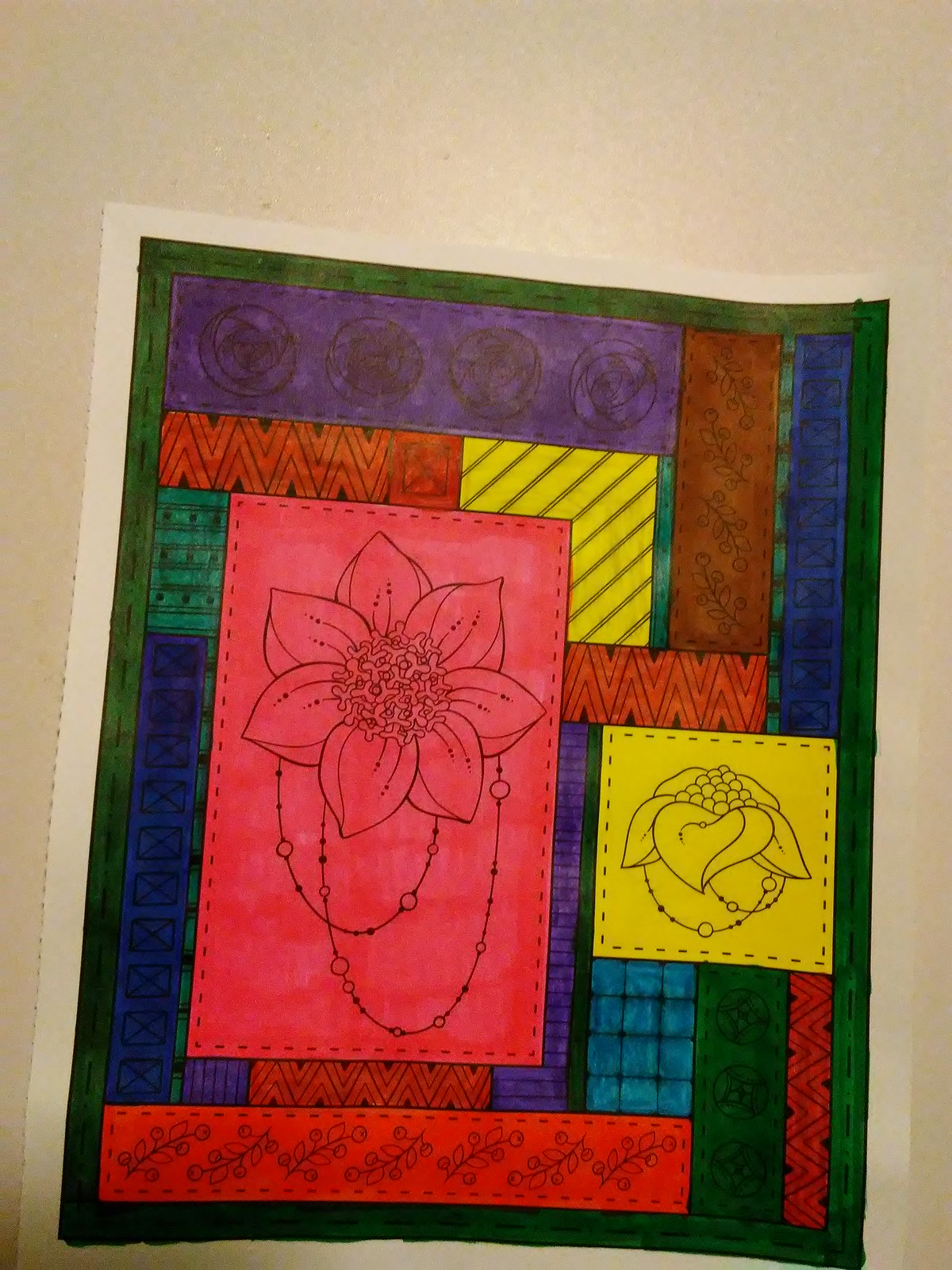This image appears to be a detailed coloring of a patchwork quilt, possibly done on fabric rather than a standard coloring book page, owing to its textured background in shades of gray, beige, and tan. The quilt design consists of various squares and rectangles, each vividly colored and patterned. It's predominantly done in markers, evident from the visible stoke lines that create varying shades where the marker overlapped. 

The border features a green scalloped edge with black dashed lines resembling stitching, further enhancing the quilt-like appearance. Within the quilt, the most prominent patches are two large squares: a left red flower with pointed petals, resembling a sunflower adorned with bead-like strands around its petals, and a right wilted yellow flower encircled by two chains, possibly depicting necklace beads.

Other patches exhibit a wide color spectrum, including purple, blue, light blue, orange, green, and brown. Notable patterns consist of a purple and yellow patch with black diagonal lines, a red zigzag pattern with black accents, and a bluish-green patch with double skinny lines interspersed with three dots. Additionally, one patch features an X in a sequence of rectangles shaded in black and purple, while another displays a box with twelve turquoise squares. Moreover, there is a rectangle filled with three rows of squares, colored green, and a design of corn with necklace beads on a yellow background. The entire image is framed by a green-bordered piece of paper, further emphasizing its intricate and vibrant design elements.